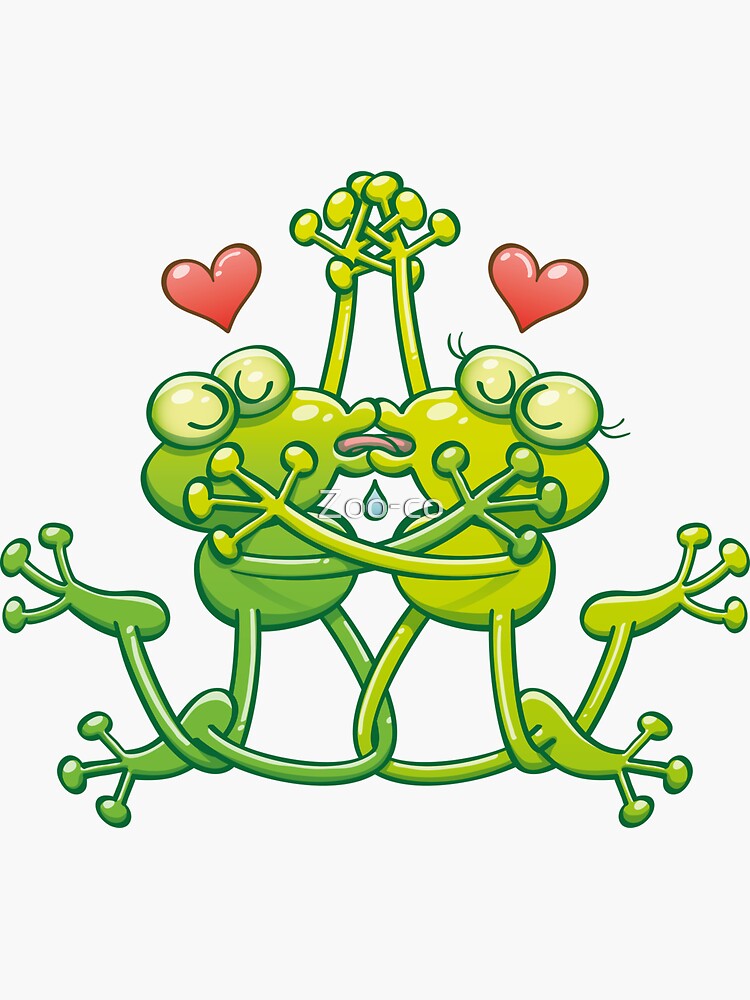In a vertical-rectangular cartoon image, two frogs are depicted facing each other in an affectionate embrace. The frog on the left is a darker green color, while the one on the right, characterized by eyelashes, is a lighter green, implying she is female. Both frogs have their mouths open with their tongues extending and touching each other, creating the effect of a passionate kiss, accentuated by a drop of drool beneath their tongues. Their front paws are touching and intertwined at the top, while their other arms are raised and embracing each other in the background. The frogs' legs are also entangled together in the center of the drawing. Above their heads, two red heart shapes float, symbolizing their love. There is white text, possibly a copyright notice, situated beneath the frogs, in front of the drool.